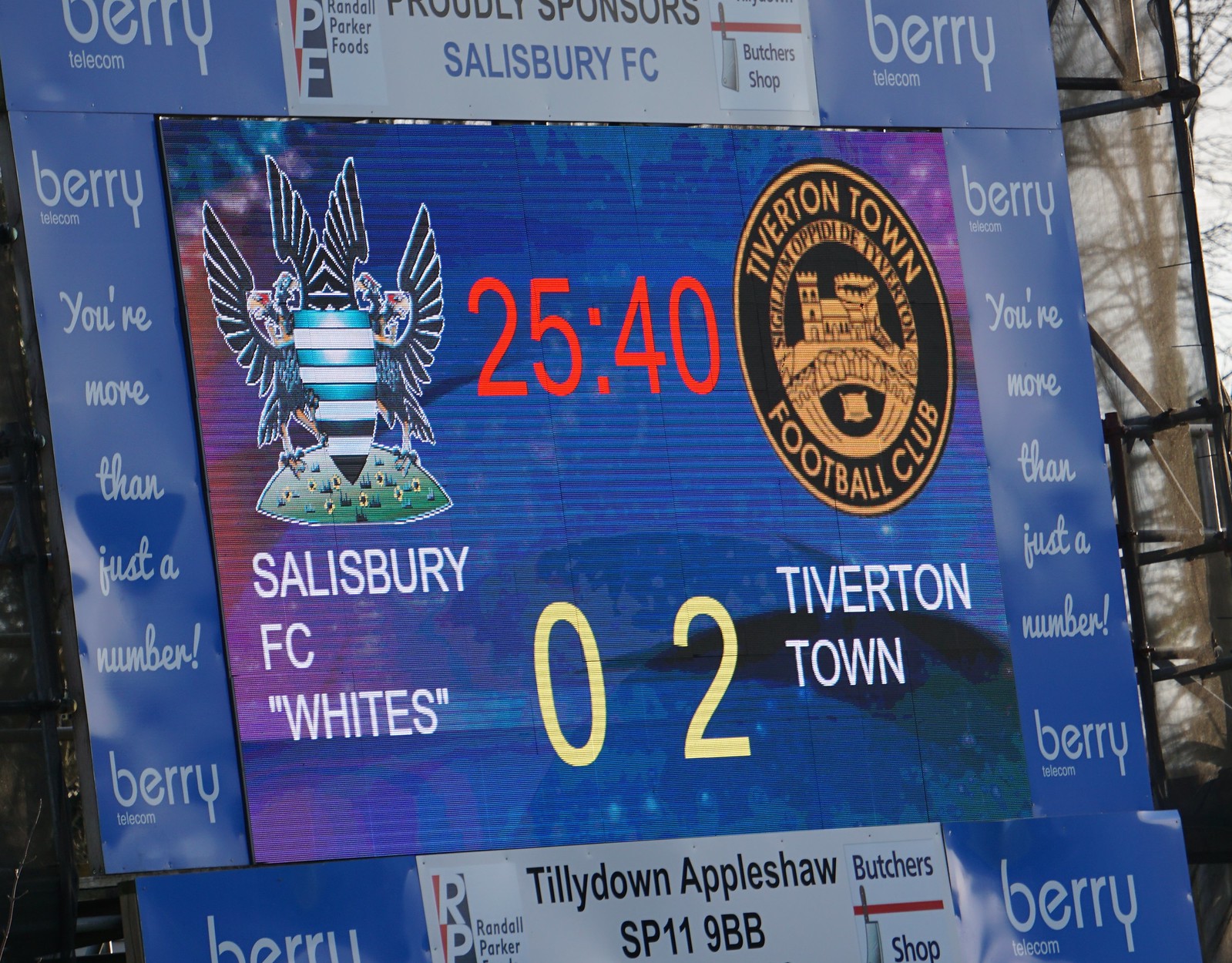The image is of a square-shaped blue scoreboard for a football match between Salisbury FC and Tiverton Town, prominently sponsored by Bury Telecom. At the top of the scoreboard, "Proudly Sponsors" is written in black, followed by "Salisbury FC" in blue. The logos of the two football clubs are displayed in the center; on the left is the Salisbury FC logo featuring blue, white, and black stripes with eagle wings, and below it, "Salisbury FC Whites" written in quotation marks. To the right is Tiverton Town’s logo, a black and gold circle with a castle and a Latin motto.

In the digital display section, the time is displayed as "25:40" in red digits, with the score "0-2" in yellow beneath it, indicating Tiverton Town is leading. On the edges of the board, the phrase "You are more than just a member" is written, reinforcing the sponsorship by Bury Telecom, featured at multiple points around the border. Along the bottom of the scoreboard, additional sponsors like Randall Parker Foods and Tilly Down Apple Shawl SP-119BB are mentioned. The outdoor setting suggests it's daytime with trees visible in the background. The unified vivid blue and occasional purple tones, combined with precise digital timings and detailed football club logos, make the scoreboard eye-catching and informative.